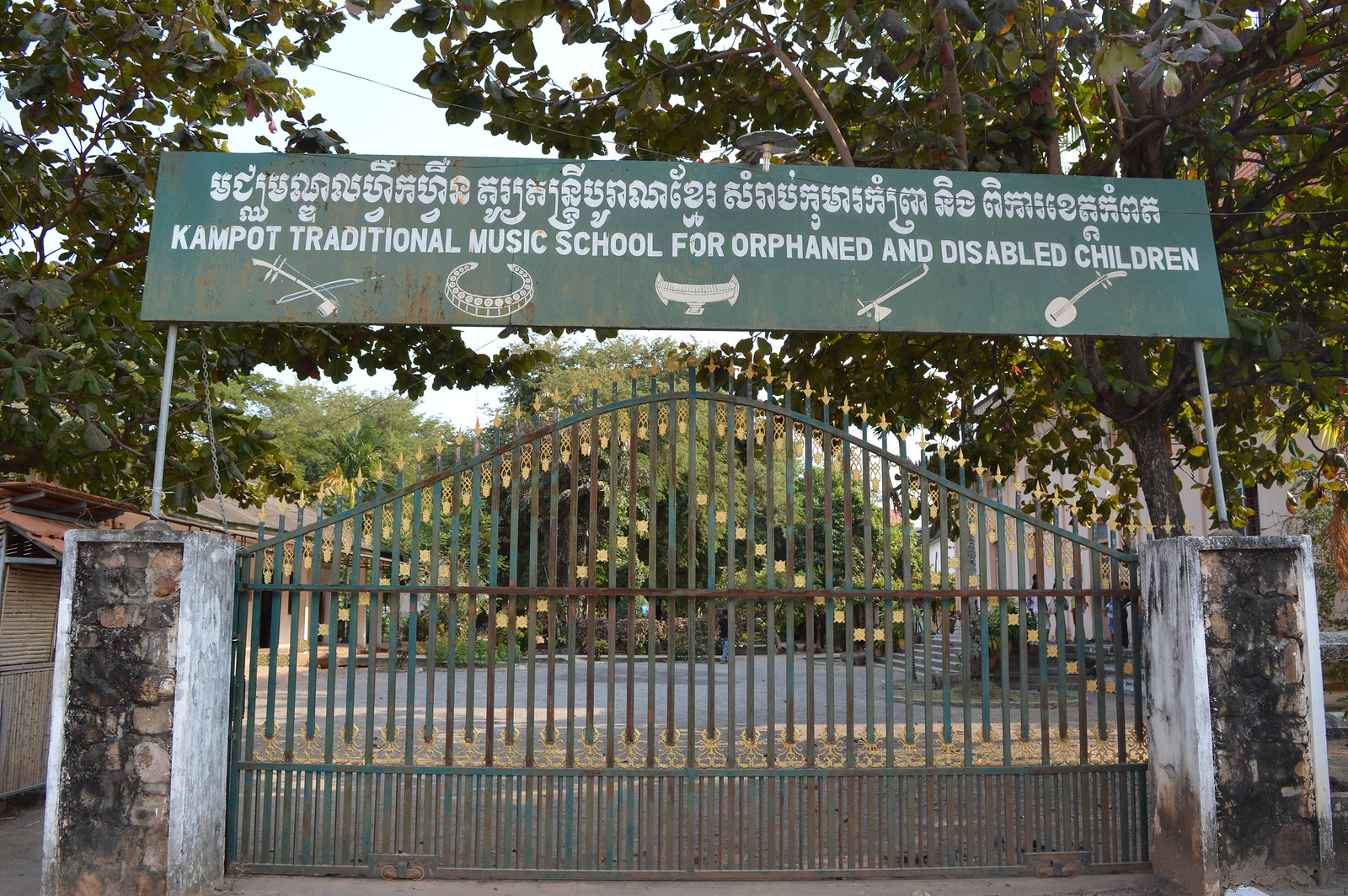The photograph captures a closed, large metal gate, flanked by two stone columns on either side. The entrance punctuates the boundary of a spacious courtyard that leads to various low-lying buildings and an expanse of trees. The metal gate features intricate design elements, including a rusty horizontal bar across the middle and a bottom section resembling a grate. Poles rise from both stone columns and join at their tops, supporting a prominent green sign. This sign has two lines: the first in a foreign language, and the second in English, reading "Kampot Traditional Music School for Orphaned and Disabled Children," accompanied by illustrations of musical instruments. The scene beyond the gate is devoid of people or cars, suggesting that the site, likely a music school for orphaned and disabled children, is currently closed.